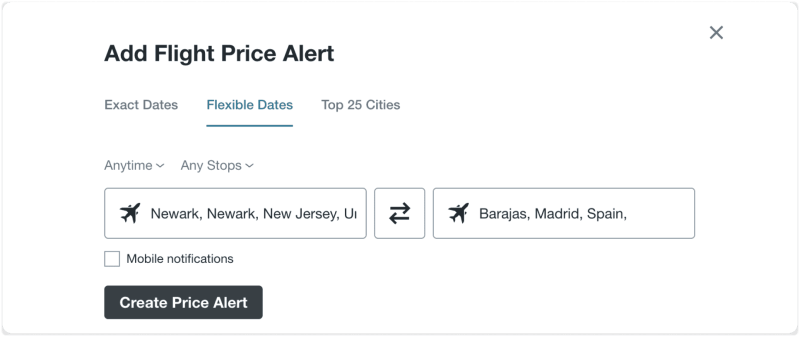A screenshot from a travel website displays a flight price alert feature. The interface offers three main options: "Exact Dates," "Flexible Dates," and "Top 25 Cities," with "Flexible Dates" highlighted in blue and underlined. Below, dropdown menus labelled "Any Time" and "Any Stops" are available for further filtering. A search box is pre-filled with a flight route from Newark, New Jersey (EWR) to Barajas, Madrid, Spain (MAD), with a plane icon between the destinations indicating the travel direction. The option to switch departure and arrival locations is implied by arrows. Adjacent to the search box is a checkbox for enabling mobile notifications, which is currently unchecked. At the bottom, a black "Create Price Alert" button with white text is featured prominently. An "X" button in the upper-right corner suggests the ability to close the window. Overall, this interface seems designed to notify users of price changes for selected flight routes.